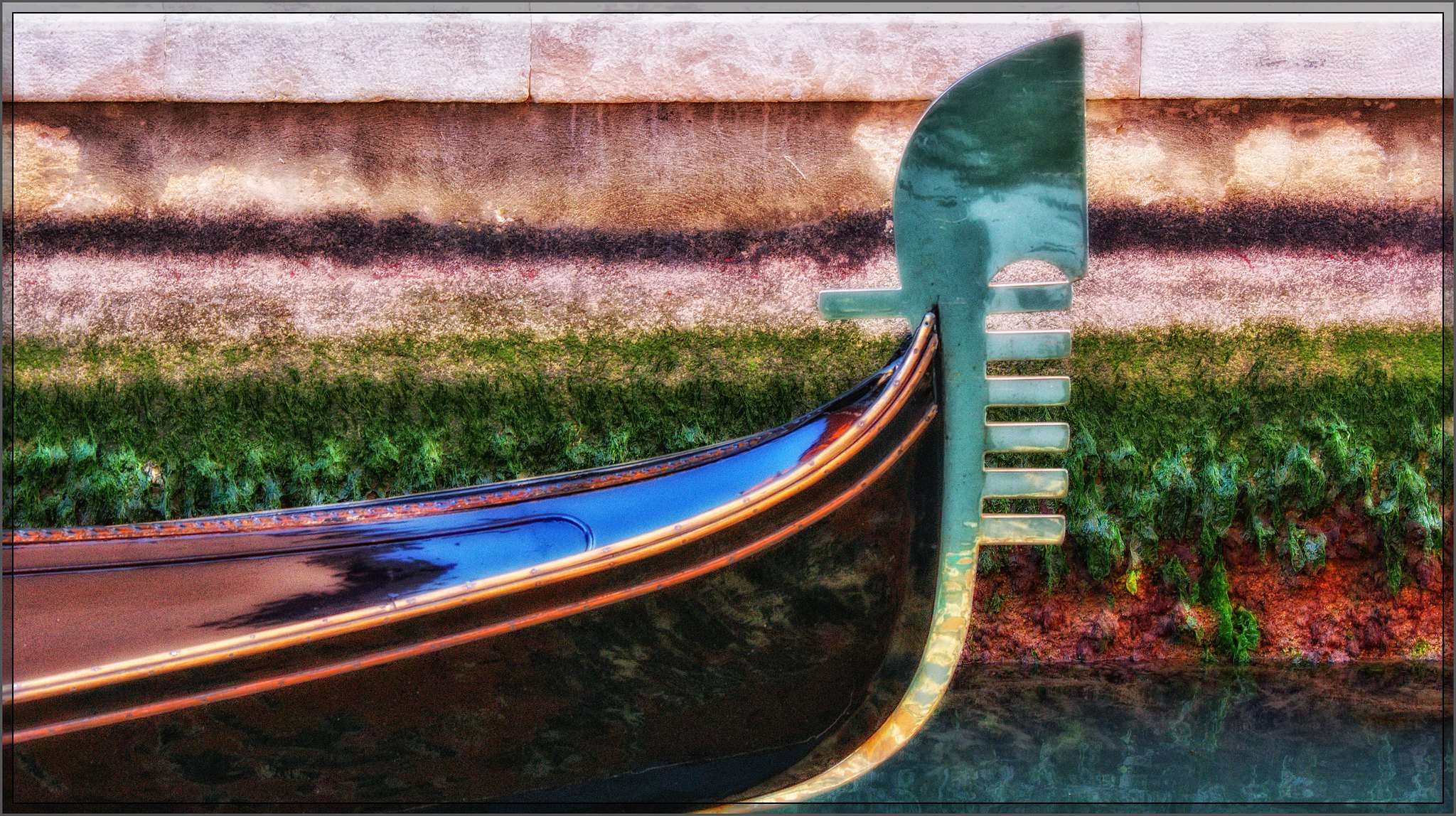This horizontal, rectangular image appears to be a detailed painting of the front tip of a small gondola-like boat, possibly set in a canal reminiscent of Venice. The gondola is predominantly black with orange striping, and its interior is blue. The bow of the boat curves upward into a point, adorned with an intricate, axe-like metal figure—resembling a blade at the top—colored in blue steel with yellow and green tints. Beneath this emblem are six horizontal bars, evenly spaced and jutting out downward. The background showcases a scenic outdoor setting with a canal wall consisting of green bushes and a weathered, pinkish-red brick wall with black streaks. The water depicted is blue, reflecting the picturesque, tranquil environment.